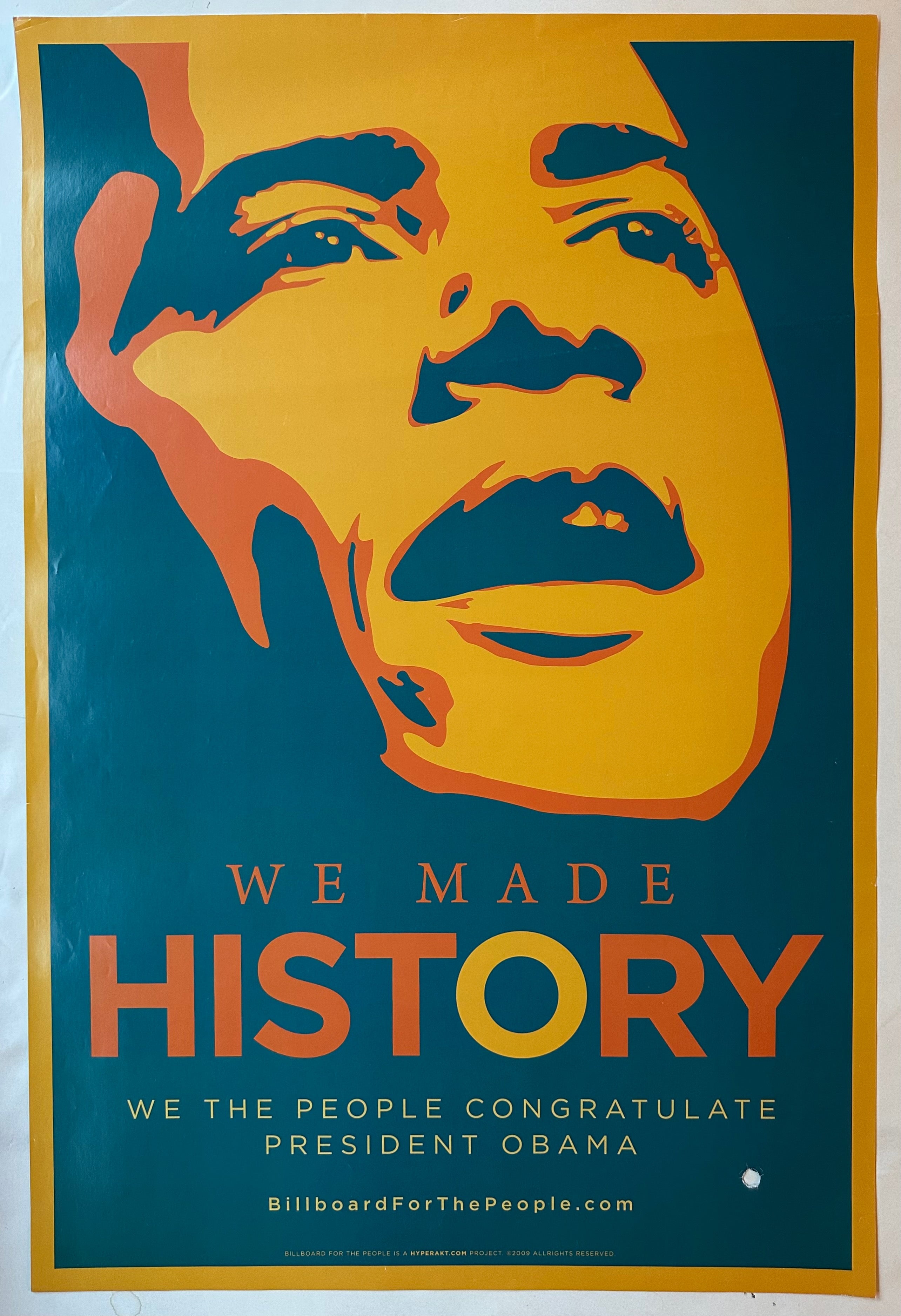The poster features an artistic, mask-like rendition of President Barack Obama's face, prominently displayed in orange and mustard hues. The silhouette of his eyes, nose, and mouth is accentuated by dark shapes. Below this evocative image, bold orange text declares, "We Made History," with the 'O' in 'History' highlighted in mustard to symbolize the 'O' in Obama's name. Underneath, in smaller print, the message reads, "We the People congratulate President Obama," followed by the URL, billboardforthepeople.com. The entire poster is bordered by a gold frame and is pinned to a white wall on one corner, either the bottom left or bottom right.